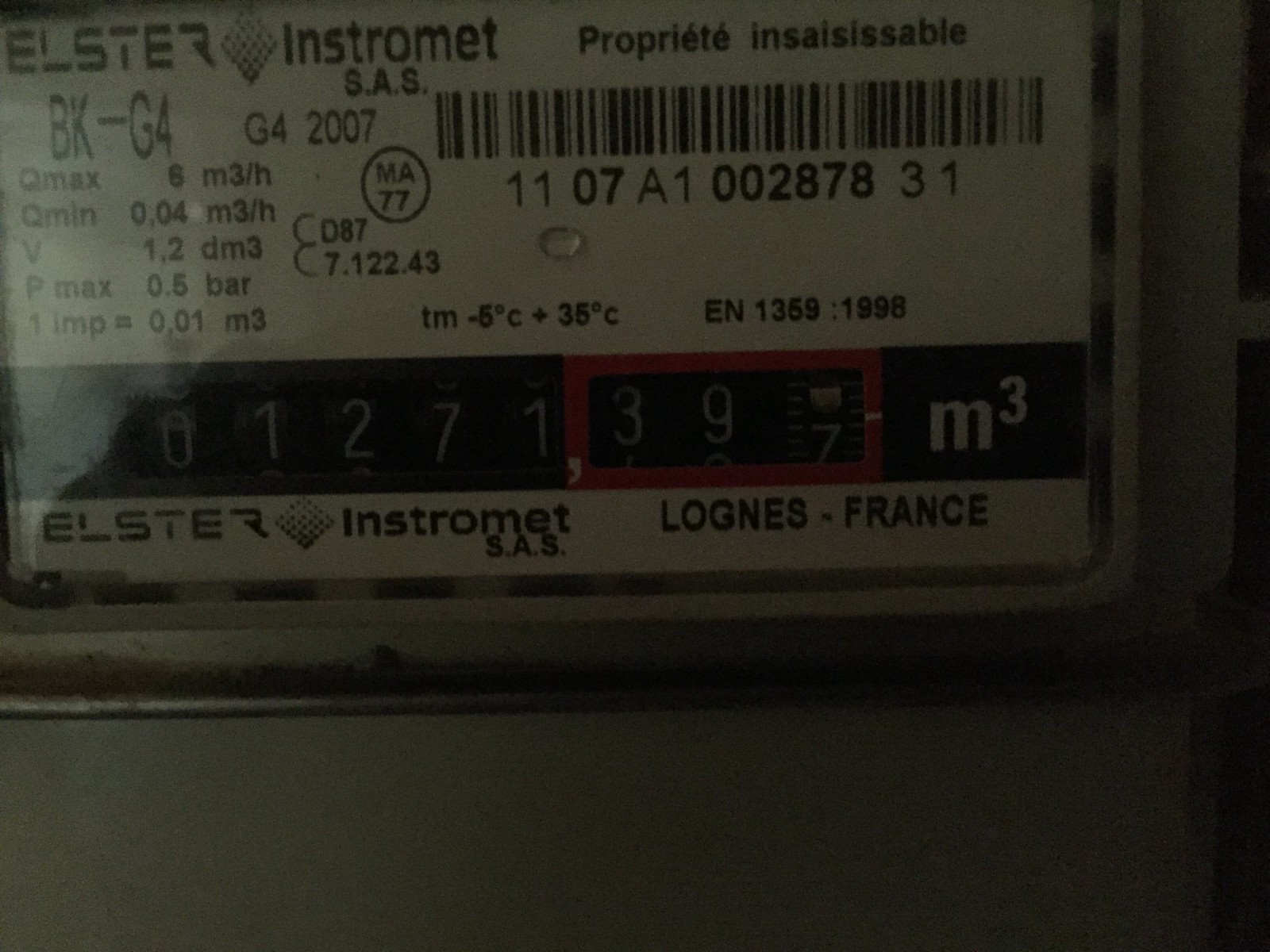The image is a detailed photograph of an informational panel and meter, encased in a clear acrylic plastic cover and mounted on a white wall. The main panel is predominantly white, displaying black text and several sets of numerical figures. At the top of the panel, the text reads "ELSTER INSTROMET SAS" with a diamond shape logo nearby and additional foreign words, including "LOGNES - FRANCE." Below, the label "BK-G4 G4 2007" and "QMAX 6 M3-H QMIN 0.04 M3-H V1,2 DM3 PMAX 0.5 BAR 1 IMP 0,01 M3" are prominently displayed. Towards the bottom of the panel, a barcode is present, above which reads the number "1107A100287831." 

A column on the left side of the panel lists various figures and data points. The meter contains black adjustable numbers, resembling old gas pump counters, which read "101271397 M3" in a segmented strip at the bottom. Throughout, the intricate design and numbers are displayed in precise black font against the structured layout of the white backdrop, providing detailed technical information about the instrument.